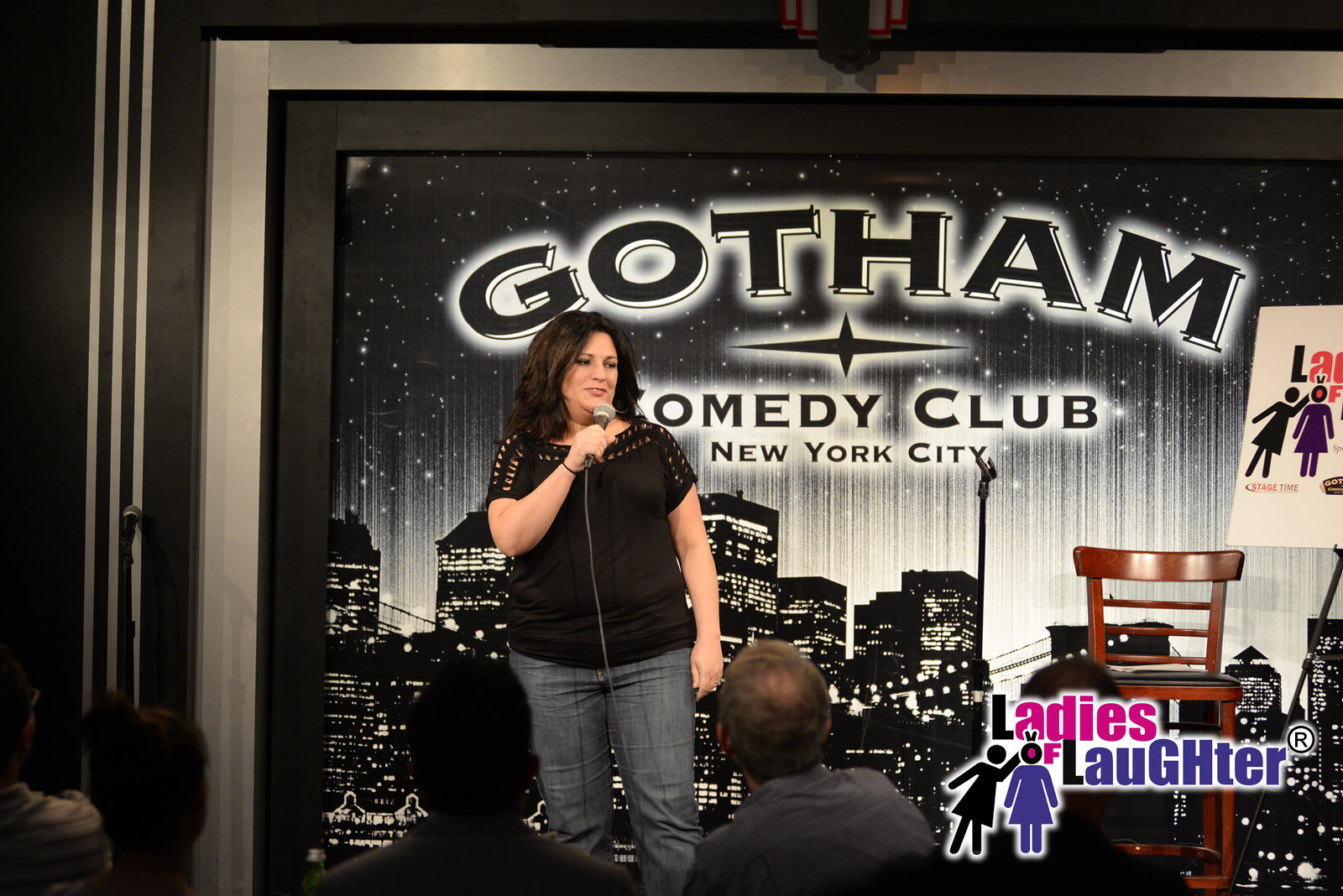The photograph captures an indoor comedy event at the Gotham Comedy Club in New York City. At the center of the image, a female comedian is standing on stage, engaging with the audience while holding a corded microphone up to her mouth with a smile on her face. She is dressed in a short-sleeved black top with a lacy fringe at the shoulders and collar, paired with blue jeans. Her long dark hair cascades over her shoulders. The backdrop features a black-and-white city skyline silhouette with lit-up windows and a starry sky above, prominently displaying "Gotham Comedy Club, New York City." In the foreground, the backs of several audience members' heads are visible, all focused on the comedian. Notably, a tall brown wooden chair and a microphone stand are positioned to her right on the stage. In the bottom right corner of the image, a logo reads "Ladies of Laughter," accompanied by icons of two women, one in black and the other in purple, with the black figure holding up her hand behind the purple one’s head.